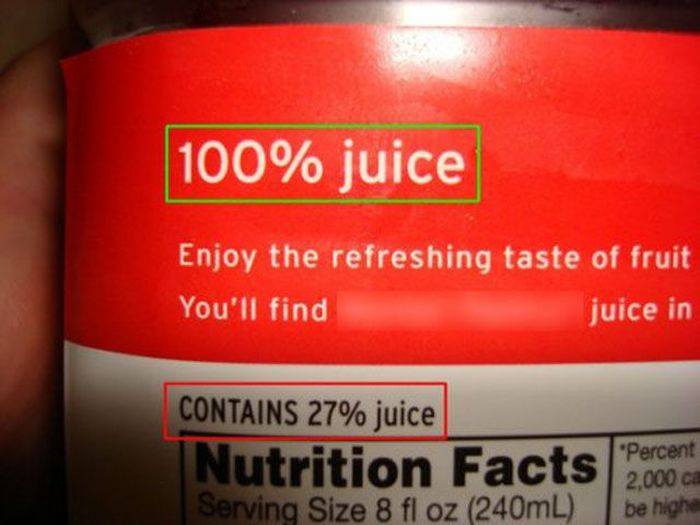This image shows the back label of a container, possibly a can or a bottle, with distinct red and white sections. At the top of the label, enclosed in a yellow box, are the words "100% juice" in white lettering. Below this, the phrase "Enjoy the refreshing taste of fruit you'll find" is partially visible but blurred out in the middle. The text continues with the word "juice in." Further down, the label states "Contains 27% juice," highlighted by a red box. This is followed by the "Nutrition Facts" section, which provides information for a serving size of 8 fluid ounces (240 milliliters). The label features a metal ring at the top edge, indicating it might be a can. The visible part of the nutrition facts includes some obscured percentages, likely related to a 2,000 calorie diet.